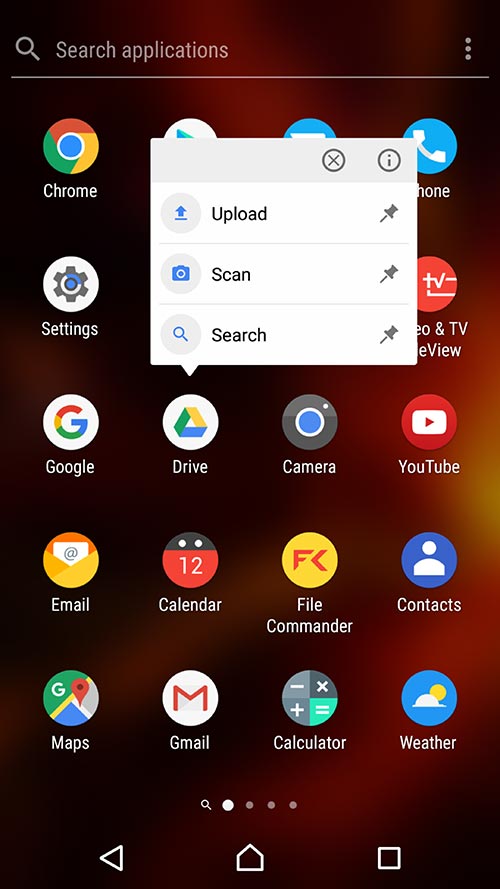The image is a screenshot of the main menu on an Android device, capturing the app drawer where users can search for installed applications. At the top of the screen, a semi-transparent search bar overlays the phone's wallpaper. Within the search bar, the phrase "Search applications" is displayed alongside a magnifying glass icon on the top left corner, signifying the search function.

The central portion of the image showcases a grid layout of app icons, arranged in a 4 by 5 format, resulting in a total of 20 visible applications. Noteworthy icons include a weather application represented by a white cloud and yellow sun located in the bottom right-hand corner, adjacent to a calculator app featuring arithmetic symbols (minus, multiply, equal, and plus). Other recognizable apps such as YouTube, Chrome, and Settings are also visible.

At the bottom of the screen, indicators show four pages of applications, with the current view focused on the first page. Beneath this, the navigation bar presents three primary buttons: from left to right, a back key, a home key, and a menu/options key. This detailed layout reflects a typical user interface on an Android device's app drawer.